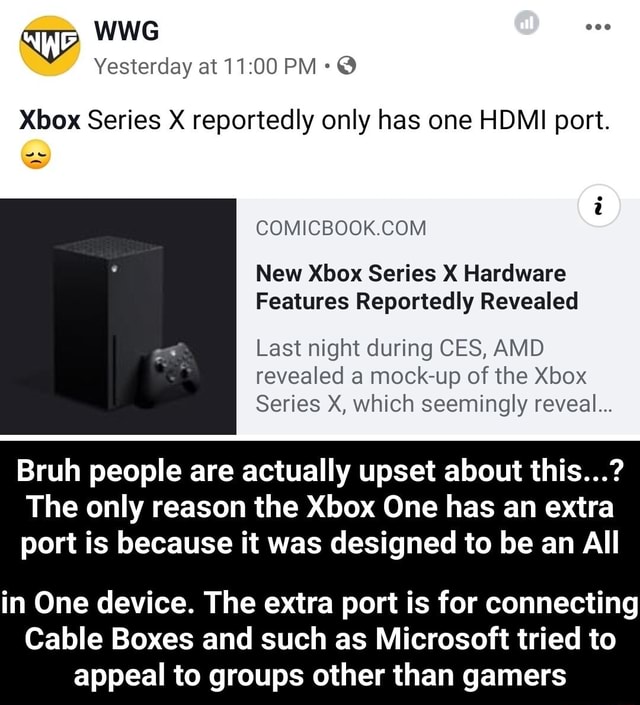This is a detailed screenshot from an unknown source. At the top, a yellow circle with the initials "WWG" in white letters is prominently displayed. To the right of this circle, there is a textual indicator that says "WWG, yesterday at 11pm." The headline announces, "Xbox Series X reportedly only has one HDMI port," followed by a sad face emoji. Below this headline, a photograph features a sleek, black Xbox Series X gaming console with a matching black controller resting against its side. 

A link to an article on comicbook.com is included, displaying the title, "New Xbox Series X hardware feature is reportedly revealed." The article mentions that "Last night during CES, AMD revealed a mockup of the Xbox Series X, which seemingly reveals..."

At the bottom, commentary is added stating, "bruh, people are actually upset about this. The only reason the Xbox One has an X port is because it was designed to be an all-in-one device. The X port is for connecting cable boxes and such, as Microsoft tried to appeal to groups other than gamers."

Notably, the image contains no people, animals, birds, plants, flowers, trees, automobiles, helicopters, airplanes, or trains.